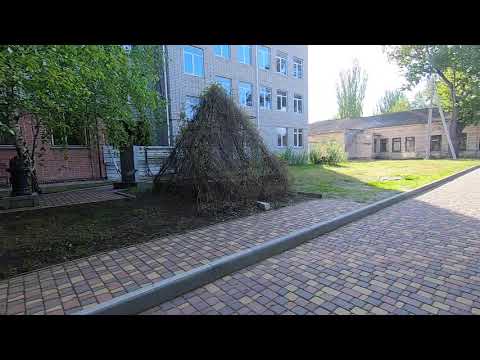This photograph captures a daytime scene of a multi-story gray stone building with numerous windows, likely indicating an institutional setting such as a college administration building. The foreground features a brick pathway composed of red, yellow, and gray bricks, flanked by a concrete curb. Among the pathway and nearby sidewalk, a notable pyramidal structure made of brown, dry wooden sticks stands out, surrounded by patches of greenery. Adjacent to this structure grows a tree within the walkway area. Additionally, a small one-story building and several green-leaved trees are visible within the property. In the background, hints of ongoing work can be observed, including a ladder against another building. The top and bottom of the image are bordered by black framing, which adds a distinct outline to the photograph. The sky above is clear, enhancing the bright atmosphere of the scene.